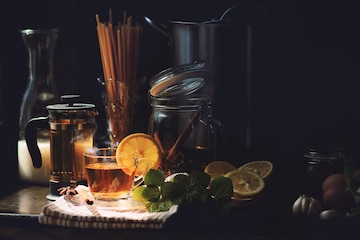This dark and moody image depicts a meticulously arranged beverage and kitchen setup on a dark-colored table. On the left side, a small clear glass containing a slice of lemon and a dark liquid, possibly tea, is perched in front of a tea diffuser container. Adjacent to it is a mason jar with a sealing lid, holding two cinnamon sticks. Behind the tea setup is a carafe filled with milk. In the middle of the table stands a unique glass bowl filled with upright linguine noodles, lending an artistic touch to the scene. To the right of the setup, large mint leaves and several lemon slices are arranged neatly. On the bottom right, brown eggs, garlic cloves, and a glass bottle also containing milk can be seen, adding to the rustic yet sophisticated feel of the arrangement. Pot holders and a tablecloth further enhance the cozy, bar-like atmosphere of the image.